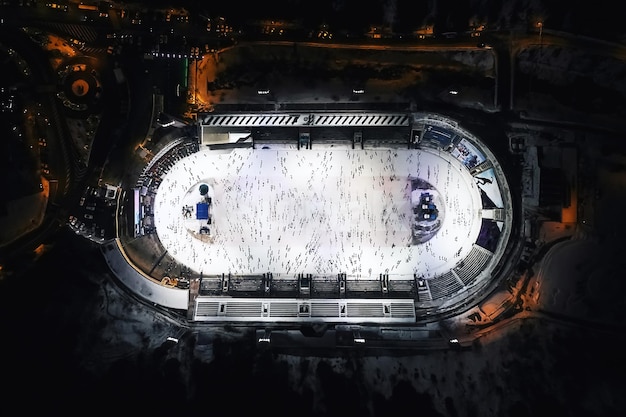This aerial color photograph, likely taken from a plane or drone, captures an elongated oval-shaped skating arena at night. The arena's ice surface, predominantly white with black streaks, is surrounded by bleachers where spectators are seated. Numerous tiny black dots on the blurred ice suggest skaters in motion. The arena is bordered by a continuous wall, and outside, the nighttime darkness is punctuated by orderly rows of streetlights, giving off soft red and yellow glows. Snow is visible around the rink, blending with the ambient illumination from the surrounding parking lots and roads. The image, unsigned and undated, also shows several indistinct blue objects positioned on either end of the rink.